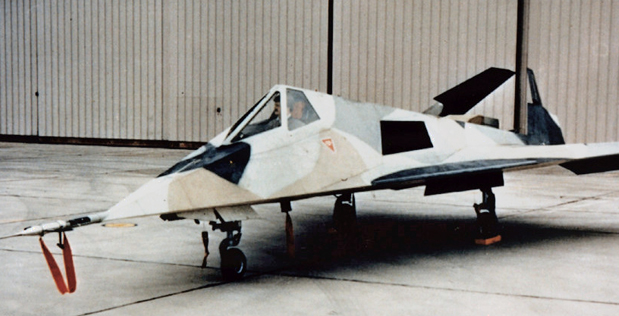This photograph showcases a small, angular stealth aircraft, reminiscent of a fighter jet, resting on a tarmac or possibly within an empty hangar. The aircraft's body predominantly features white paneling accented with black wingtips and other black areas, as well as light gray and tan shading, suggesting its design is suited for desert environments. The plane's distinct triangular shape includes a raised cockpit that slants towards a spiky nose equipped with red or orange ribbons, likely indicative of test fixtures or instrumentation pitot tubes. The tail appears slightly folded, and chocks are visible under the three landing gear wheels, affirming the aircraft is grounded. A pilot is seen inside the cockpit, seemingly conducting engine run-ups and gauge monitoring rather than preparing for takeoff. The background includes a beige-colored wall and tiled surface, further indicating a testing environment rather than an active runway.